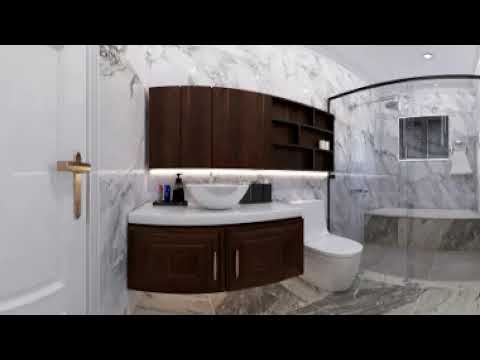The image depicts a well-designed, luxurious bathroom with extensive use of marble. The bathroom features marble walls and a marble floor with a grey pattern. On the right side, there is an elegant glass-enclosed shower, complete with a marble bench and a small window. Moving to the left, we spot a classic white toilet, positioned underneath brown wooden shelves. Further left, there is a vanity area with a white bowl-shaped sink mounted on a white marble countertop, above brown wooden cabinets. Above the vanity, more cabinets provide additional storage. The bathroom is illuminated by recessed lighting in the ceiling, highlighting the room's sophisticated color palette that includes black, white, gold, brown, tan, gray, and silver. A white door with a gold handle marks the entrance to this luxurious space.